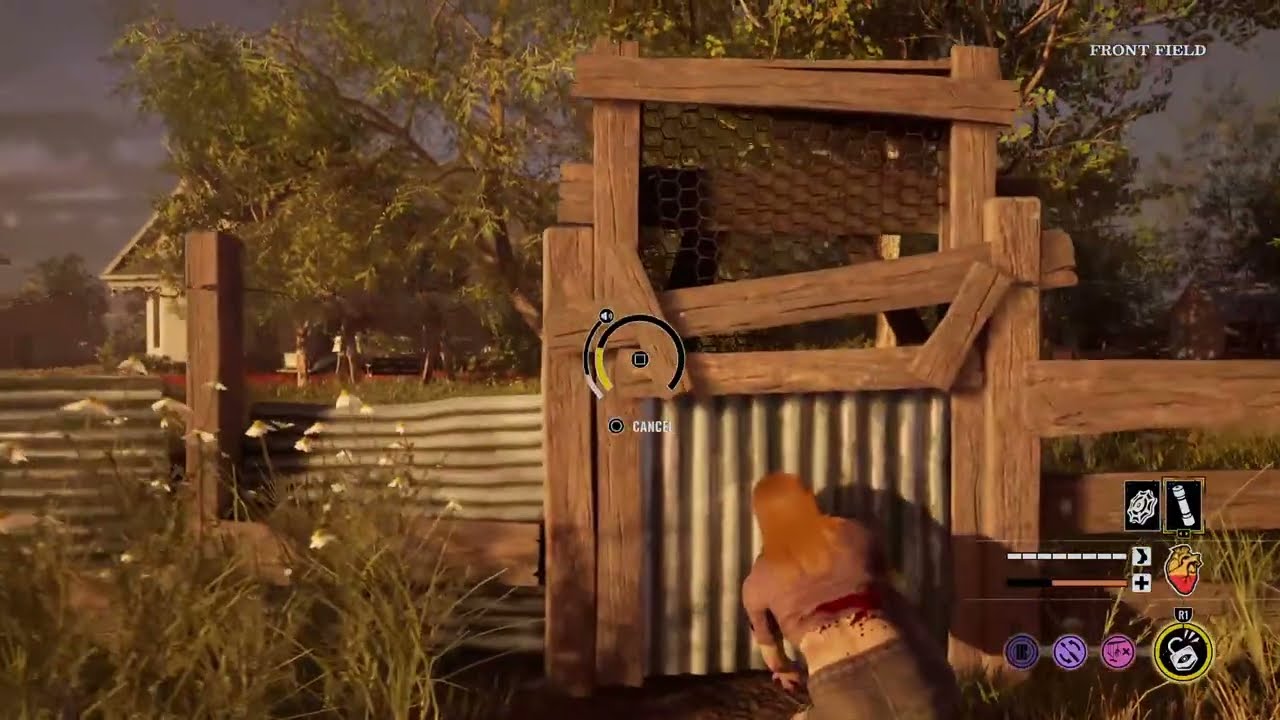The image is a screenshot from a third-person, realistic-style video game, showing a female character crouching about 4 or 5 feet in front of a slightly elevated camera. The woman, with orangish hair and clad in brown pants, seems to be hiding behind or interacting with a white farm fence, which has a brown wooden top and a corrugated metal section that may be raised to allow animals through. The scene is set in a countryside-like location with a portion of a house visible in the distance to the left and trees overhead. Small white flowers are blooming in front of the fence. The user interface in the bottom right-hand corner displays icons, including a heart, a lock, and potentially other buttons related to the character's backpack or weapons. The upper right-hand corner of the screen reads "Front Field," indicating the location in the game.